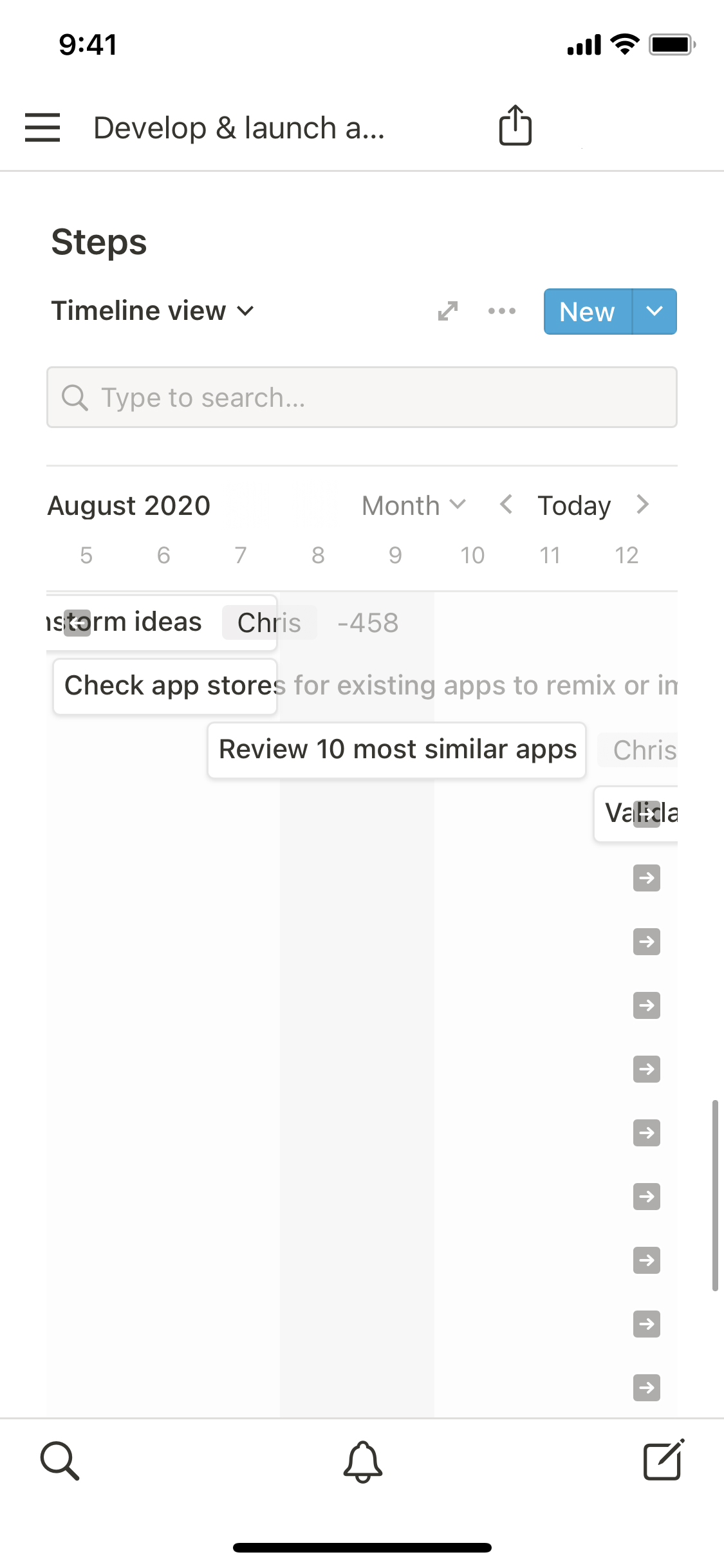The image depicts an awkwardly formatted interface, likely a mobile site rather than an app, with elements seeming ill-suited for mobile screens. The interface resembles the layout of Google Docs or Google Sheets, struggling to adapt a desktop format to mobile, causing elements to merge and appear disjointed. The screen displays words such as "steps" and "timeline view" along with a calendar set to August 2020, suggesting a record of recent events, possibly related to user activity on various applications. The background is white, adding to the overall clunky and somewhat disorganized appearance. The design inefficiencies indicate that the interface would be better suited for a desktop view.